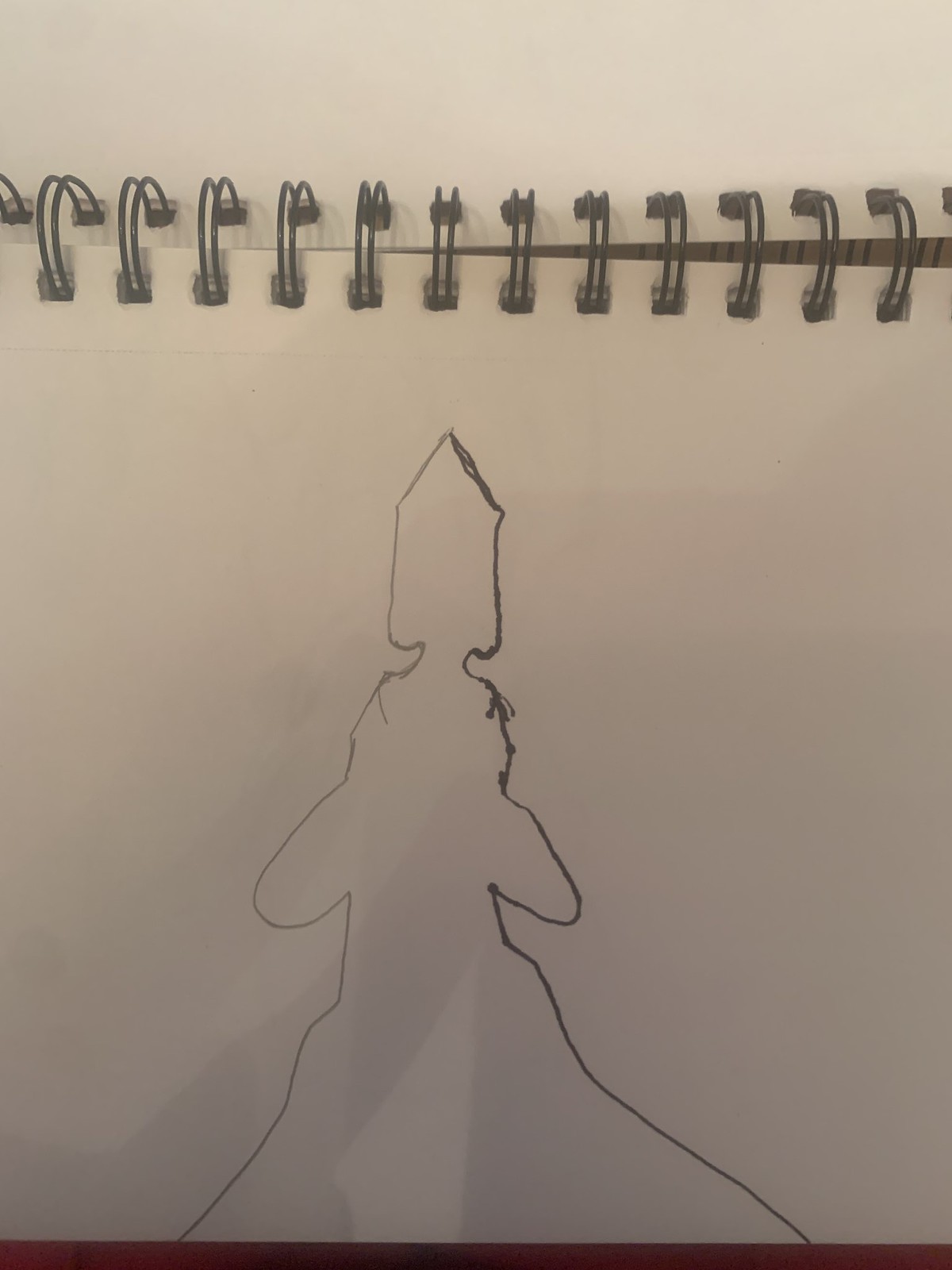This is a color photograph showcasing a small section of a page from a sketchbook positioned towards the top of the frame. The spiral binding of the sketchbook is visible, highlighting the context of the image. The sketch, a minimalist creation possibly rendered with pencil, charcoal, or ink, appears to feature a few distinct elements. At the very top of the page, there is an abstract, arrow-like figure. Below this, there's a simplistic outline that could be interpreted as the form of an animal, possibly resembling a bear or a teddy bear. Further beneath, the lines suggest the presence of arms, with the lines on either side slanting outward, creating a dynamic and abstract impression. The overall design is very rudimentary and open to various interpretations, inviting viewers to project their own meanings onto the sketch.